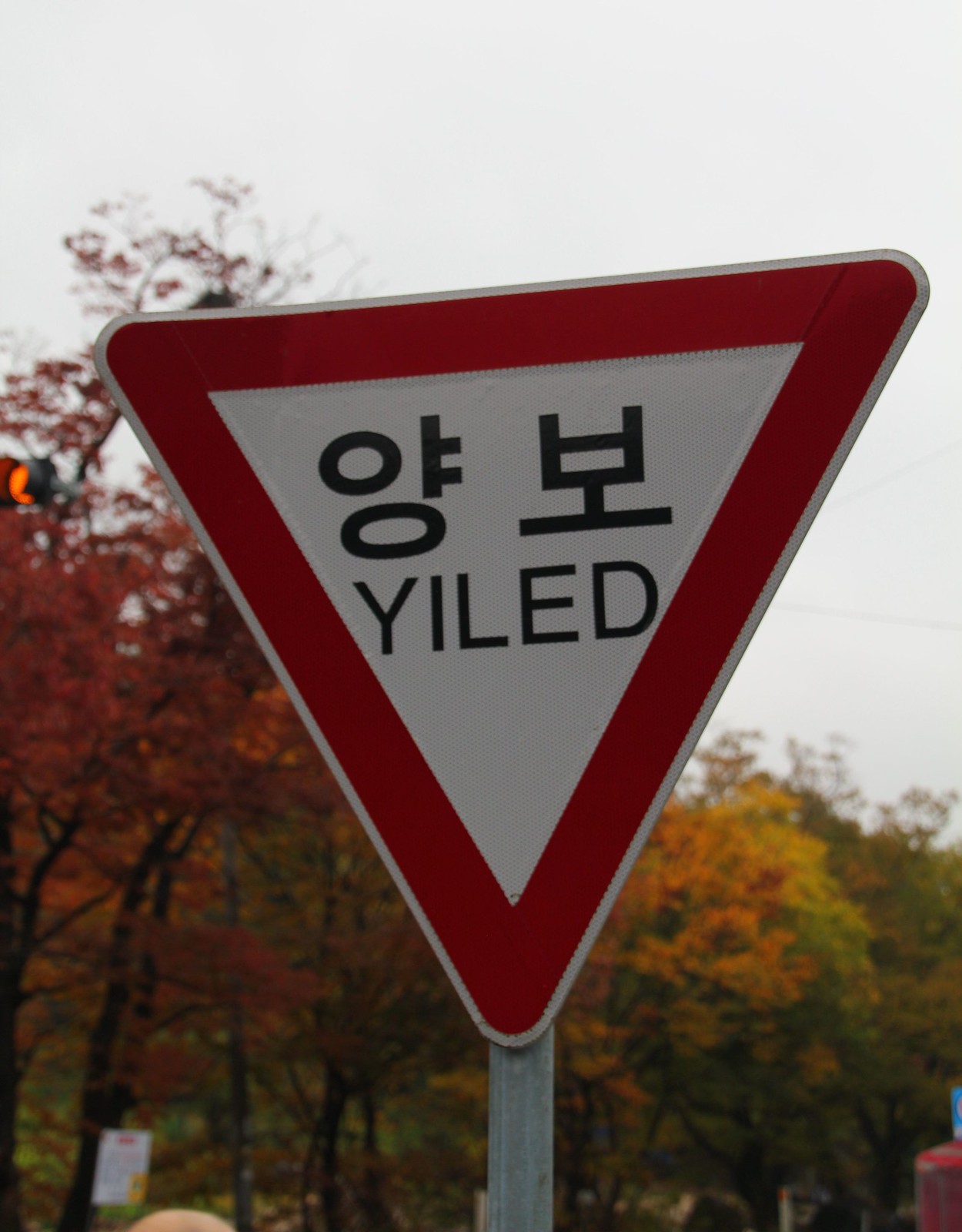This outdoor photograph captures a crisp, autumn day under a gray sky. The upper portion of the image features a canopy of slender trees adorned with leaves in vibrant autumn hues—reds, oranges, yellows, and some lingering greens. The scene conveys a chilly atmosphere. In the lower left corner, a distant, blurry rectangular white sign is visible but not legible. Central to the image is a light gray metal pole supporting an upside-down triangular yield sign, marked with a red outer border, a smaller white inner triangle, and both Asian characters and the mistakenly spelled English word "YILED" (Y-I-L-E-D). Additionally, a small, yellow light with a black border juts out to the left side of the sign, hinting at the international setting of this picturesque, fall landscape.